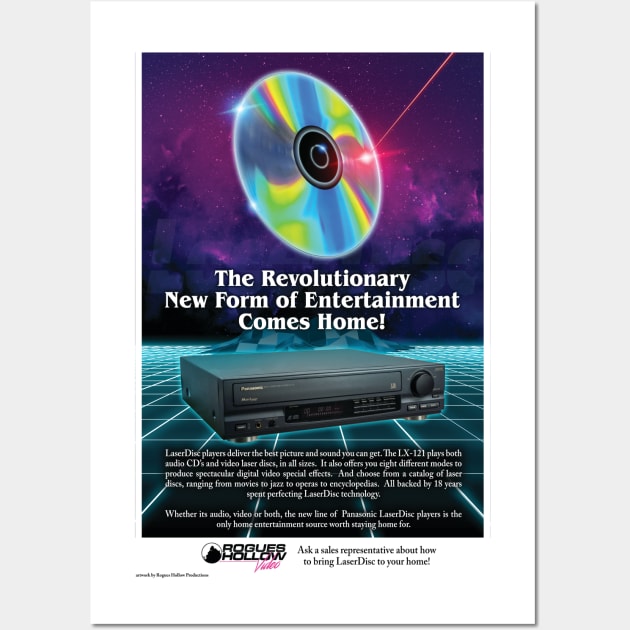This vertically rectangular advertising piece, likely a magazine page or poster, features both photographic and digital elements framed by light gray side borders and a white border encompassing the entire image. Dominating the top third of the ad is a psychedelic-colored compact disc positioned against a purple, starry sky with faint tree silhouettes. A striking red laser beam from the upper right corner hits the disc, highlighting its reflective surface. Below the disc, bold white text proclaims, "The Revolutionary New Form of Entertainment Comes Home!" A photograph of a sleek black Laserdisc player, slightly angled to the right, is situated beneath this text. Accompanying the player is a dense block of white text, too small to decipher, followed by a distinct space and two additional lines of white print. Near the bottom of the ad, within the white border, the brand name "Rogues Hollow Video" is clearly visible, alongside a note urging readers to "ask a sales representative about how to bring Laserdisc to your home."